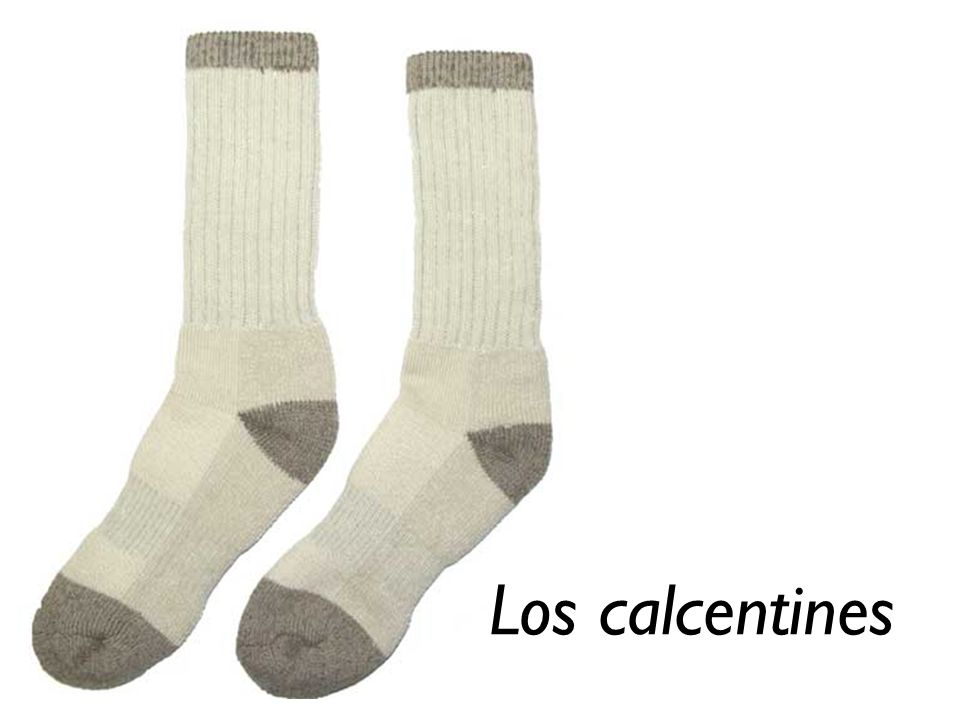The image is a product photo featuring a pair of light gray socks on a stark white background, likely intended for a website or e-commerce listing. The socks are laid side by side, slightly angled to the left, with one sock's toe pointing towards the bottom left corner. Each sock has a dark gray toe, heel, and a matching dark gray band at the top trim. The body of the socks is a lighter gray with visible seams and subtle speckled patterns adding texture. Alongside the socks, in the bottom right corner, there is black text reading "Los Calcentines."